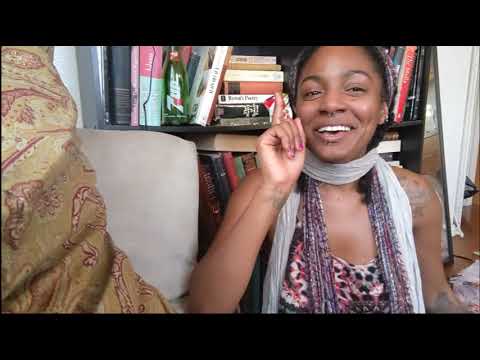The image captures an African-American woman seated in an interior setting, possibly a still frame from a video. She is shown from the chest up, with her head slightly cut off at the top. Smiling and seemingly in the midst of a conversation, she gestures with her right hand, her index finger pointing upwards. Her fingernail, painted pink, adds a subtle touch of color. She wears a striking combination of scarves—one silver or gray and one purplish-black—draped around her neck. Her attire features a white, pink, and black floral print dress.

Distinctive tattoos adorn her left shoulder, left forearm, and right wrist, and she sports a nose piercing at the center of her nose. Her surroundings include a bookshelf filled with books arranged both upright and sideways, and a green 7-Up bottle, likely empty, situated on the shelves. To her right is another chair adorned with a cushion covered in black, gold, and red material. Additionally, a sideways pillow with a yellowish cover and red shapes rests on the edge of a seat beside her. The woman, caught in a lively moment of expression, sits against a backdrop that speaks to a vibrant and detailed life.